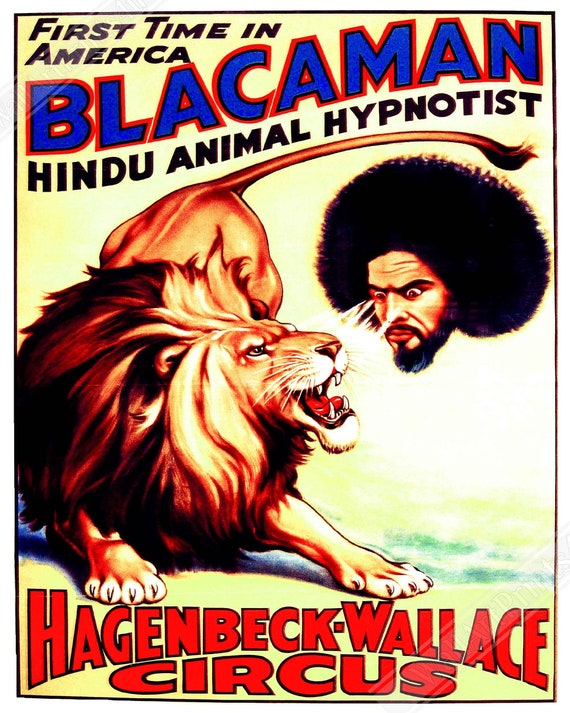The image is an old-fashioned circus poster with a predominantly pale yellow background. At the top left corner in black letters, it says "FIRST TIME IN AMERICA." Below that, in large blue block letters outlined in red, it reads "BLACK-A-MAN." Following this, in black bold letters that curve across the page, it says "HINDU ANIMAL HYPNOTIST." The center of the poster features a large male lion crouched with its mouth open, displaying its teeth, ready to pounce. The lion's tail extends towards the right edge of the poster. On the right side, a man with a huge black afro and a black beard, which includes a goatee, is intently staring at the lion. His eyes emit white beams, adding a sense of magical intensity to his gaze. Below the lion, in bright red bold letters, it states "HAGENBECK-WALLACE CIRCUS." The overall vintage look of the poster is accented with slight beige tones and a small smudge of green near the lion’s paw.